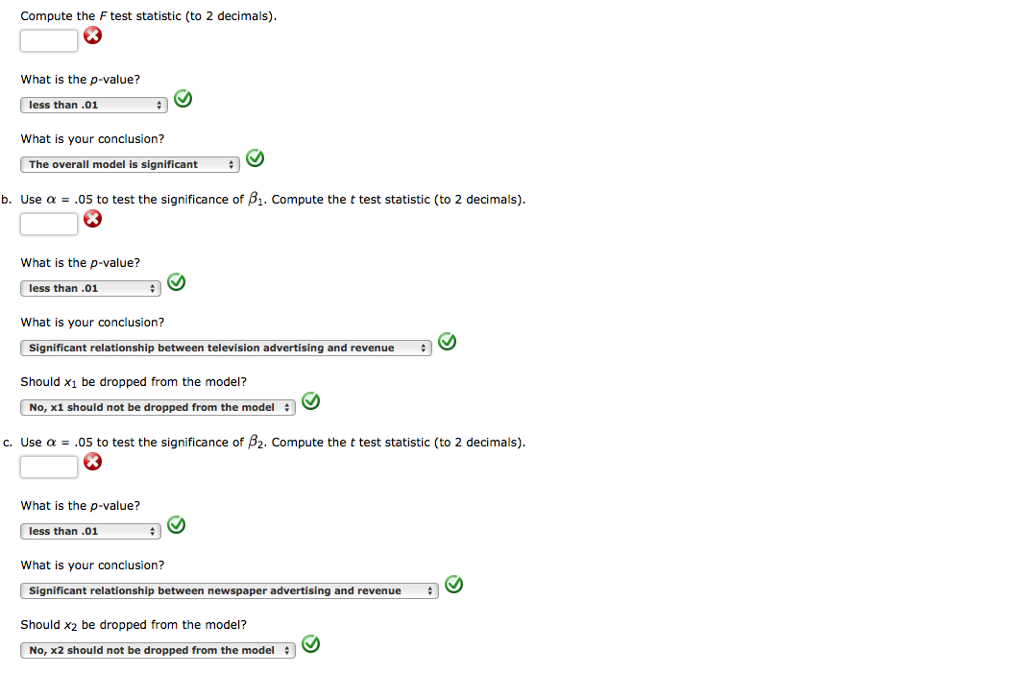In the image, we see a vertical screenshot of a computer quiz interface, occupying roughly 50% more in height than in width, set against a pure white background. The top of the quiz presents a question in black text: "Compute the F-test statistic" with a directive to provide the answer "to two decimals." This question remains unanswered as indicated by a blank space followed by a red 'X' on the right.

Below this, another question reads, "What is the P-value?", accompanied by a dropdown selection box. The selected answer is "less than .01," marked correct with a green checkmark on the right.

The subsequent query asks, "What is your conclusion?", and once again features a selection box. The chosen response, "the overall model is significant," is verified by another green checkmark next to it.

Following this section, the quiz introduces a new set of questions labeled with "B". It starts with: "Use alpha = .05 to test the significance of β1. Compute the T-test statistic to two decimals." This question, like the initial one, remains unanswered, as indicated by a blank space followed by a red 'X'.